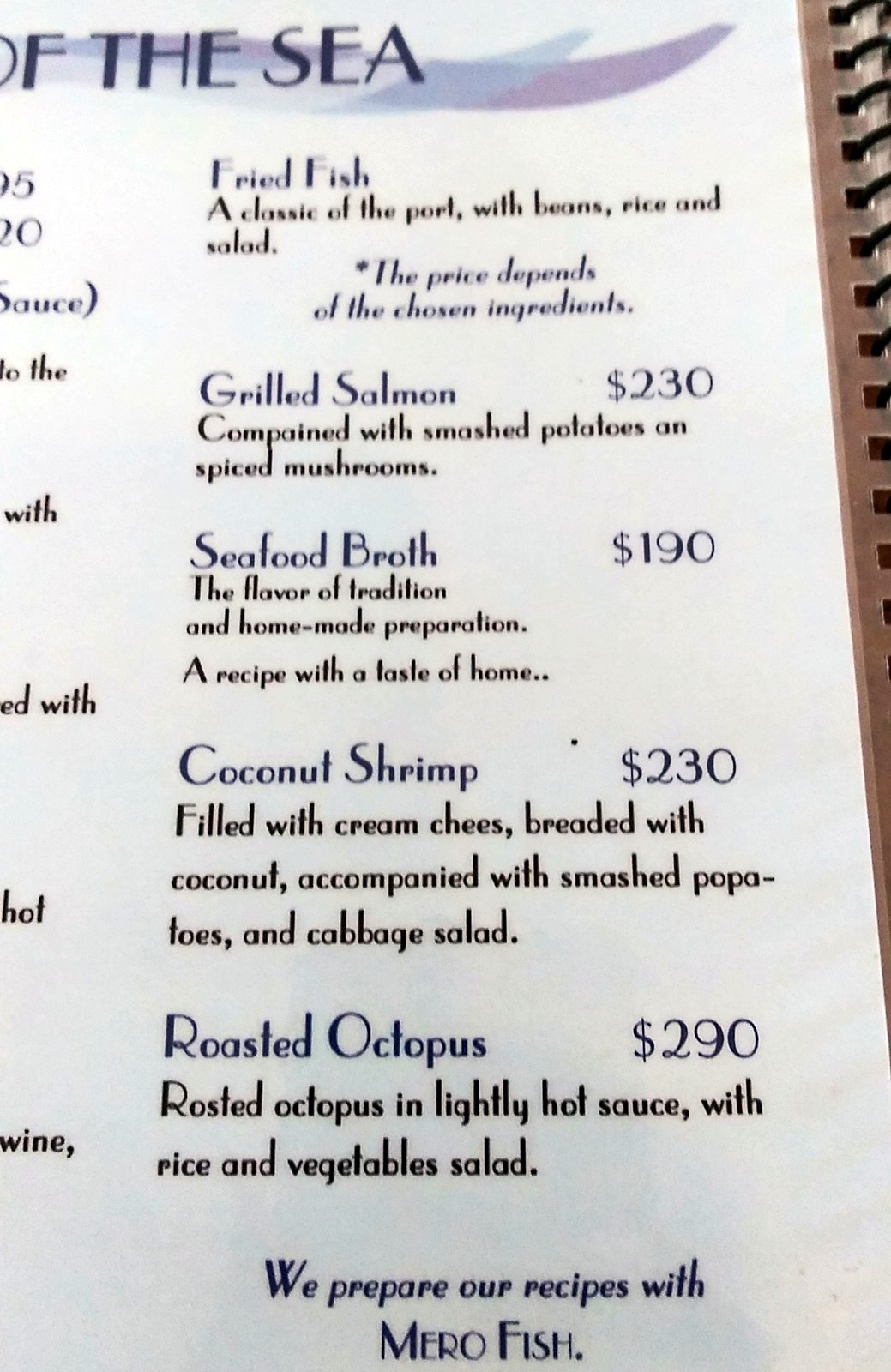Photograph Caption:

This image captures a partially visible menu from a restaurant, with the left-hand side cut off. The title or name of the establishment is seen at the top, beginning with a partial "O," followed by "F THE SEA." 

The menu items listed include:
1. Fried Fish - Described as a classic port dish served with beans, rice, and salad.
2. Grilled Salmon - Priced at $230, this dish is served with smashed potatoes and spiced mushrooms.
3. Seafood Broth - Available for $190.
4. Coconut Shrimp - Priced at $230, these shrimp are filled with cream cheese, breaded with coconut, and accompanied by smashed potatoes, papatoes (assumed to mean potatoes), and cabbage salad.
5. Roasted Octopus - Priced at $290, this roasted octopus comes with a lightly hot sauce, rice, and vegetable salad.

At the bottom, there is a note that reads: "We prepare our recipes with marrow fish."